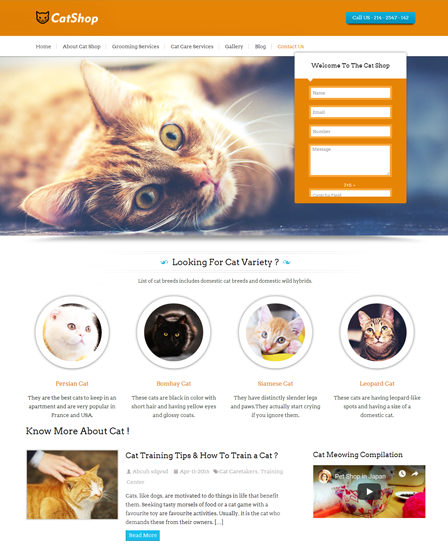The website titled "Cat Shop" features a prominent white banner at the top displaying an orange rectangle with a cat icon and the words "Cat Shop" next to it. Adjacent to this is a blue rectangle with a partially visible phone number, "Call Us: 214-2547...". The homepage includes a navigation menu with options like Home, About, Cat Shop, Grooming Services, Cat Care Services, Gallery, Blog, and Contact Us. 

A large welcome banner highlights an orange cat laying on its side, facing the viewer. Below, it reads "Welcome to the Cat Shop" followed by "Looking for Cat Variety? Our List of Cat Breeds includes Domestic Cat Breeds and Domestic Wild Hybrids." The webpage showcases detailed descriptions and images of various cat breeds, such as Persian Cats (ideal for apartments, popular in France and USA), Bombay Cats (black with short hair and yellow eyes), Siamese Cats (notable for their slender legs and tendency to cry if ignored), and Leopard Cats (domestic cats with leopard-like spots).

Additionally, the site offers extensive cat advice and tips, including sections like "Know More About Cats" accompanied by an image of an orange cat being petted, and "Cat Training Tips." A specific blog post titled "How to Train a Cat" provides training insights, emphasizing that, much like dogs, cats are motivated by benefits from their actions, involving food treats or favorite toys. At the bottom, there's a video titled "Cat Meowing Compilation" providing entertainment for cat lovers. Lastly, a contact form invites visitors to input their name, email, and message to engage with the Cat Shop team.